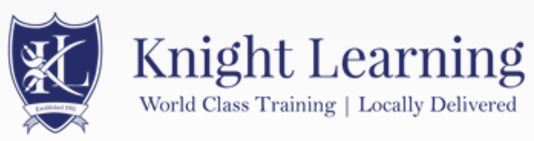The image is a low-quality, blurry screenshot of a logo for a website called Knight Learning, spelled K-N-I-G-H-T, like the English knight. The logo features a white rectangle with blue text on the right side, prominently displaying "Knight Learning" in a larger font and "World-Class Training" in a smaller font beneath it. Below that, there's the phrase "Locally Delivered." On the left side is a shield-shaped crest with a complex design. The shield has a dark blue border followed by a white border, and the inside is solid blue. The crest contains the letters "I" and "L" in white, with two crossed swords making the "I" resemble a "K," thus reading as "K L" to match the Knight Learning text. A banner at the bottom of the shield states "Established" along with an unreadable year. The overall color scheme of the text and graphics is blue and white.